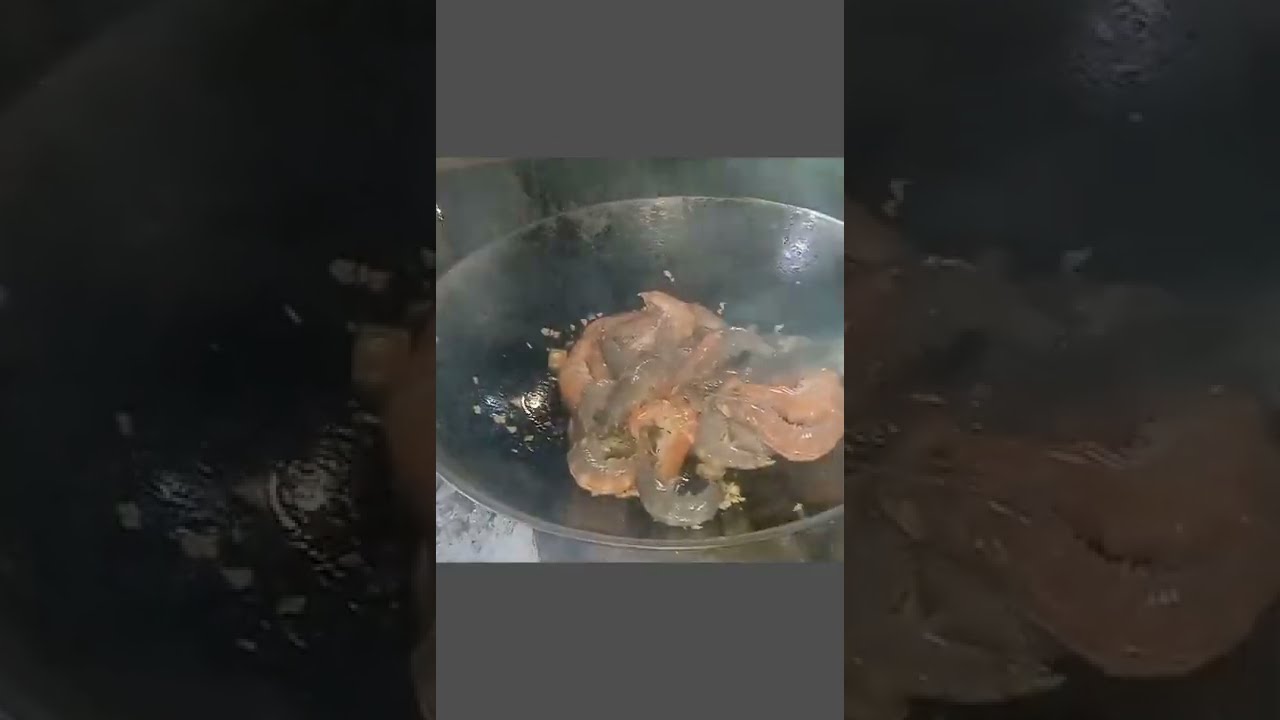In the center of this image, there is a wok-like pan with gently curved edges, containing various pieces of what appear to be raw meat. The meat exhibits a range of colors, including dark gray, pink, and reddish-brown, with some smaller bits possibly resembling chopped up onions. The pan itself has a gleam, suggesting it might contain oil, and it's situated on a metal surface that appears to have stone underneath. Surrounding the central image, there is a thick gray border on all sides, which looks like it has been grayed out and enlarged from the middle section to create a consistent frame. The overall quality of the image is poor, making finer details difficult to discern, but hints at a mobile device screenshot given the orientation and framing. There is no text present in the image, and the colors are primarily shades of gray, white, pink, and black.